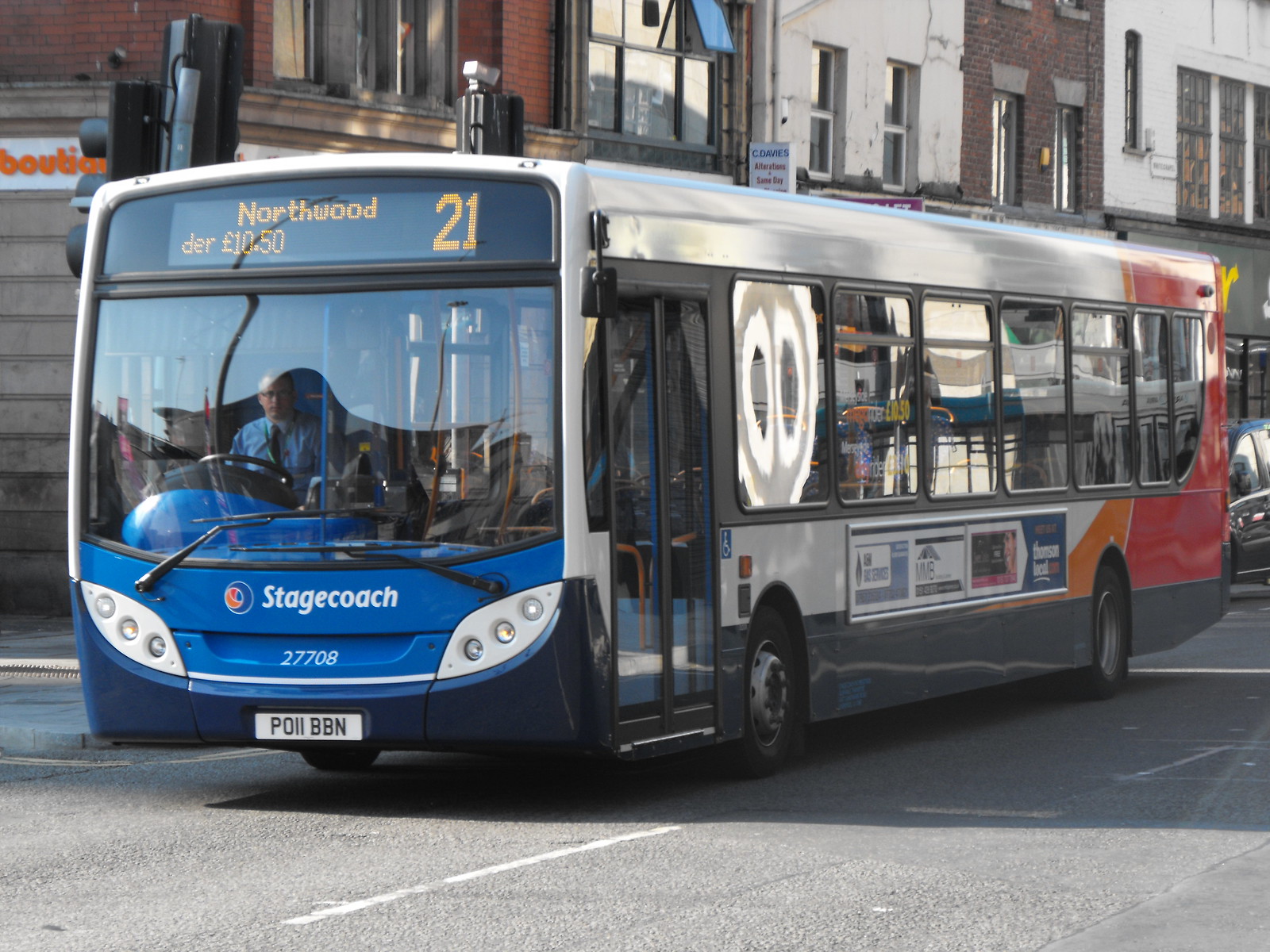In this image, you see a public transit bus driving across a city street, captured from an angle that reveals both its side and front. The bus is distinctive with its white, blue, red, and orange color scheme. Its front displays the route information "Northwood 21" and "Northwood DER L10.50". Below the windshield, the label "Stagecoach" is printed, along with the number "27708". The bus features three headlights on each side of its blue front section, and the license plate reads "POIIBBN".

In the large front window, the bus driver is visible, wearing a tie and a blue shirt. The left side of the bus has big windows and black doors, with unreadable advertisements in the lower middle section. The rear of the bus is red and orange, further adding to its multicolored appearance.

The background features a mix of red brick and white-colored buildings, likely apartment complexes, standing two stories high. The image is slightly blurred, suggesting motion, with the bus seemingly in mid-transit on a typical city street.